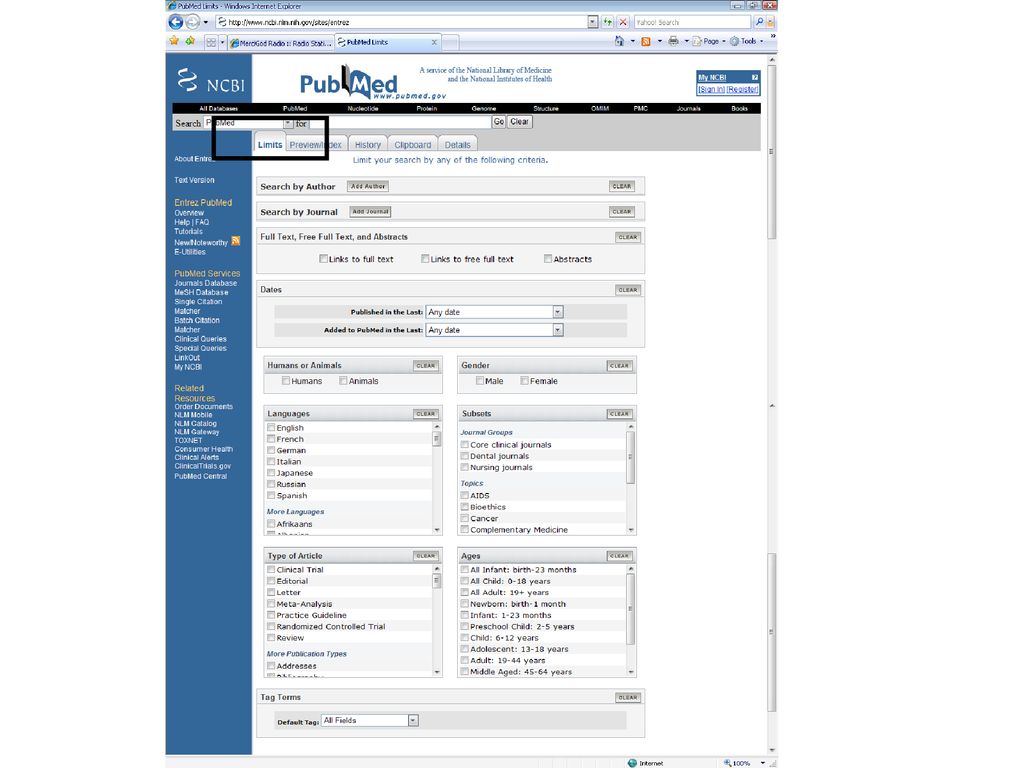The screenshot captures the PubMed website displayed in an Internet Explorer browser. The web address in the browser's address bar shows "NCBI," indicating the site being accessed is indeed PubMed. At the top of the interface, a black horizontal menu bar features white font, and it appears to encase various website options.

Below the general menu bar, two search bars are aligned side by side, positioned just above another black bar labeled "Limits." This section includes tabs for navigation—"Limits," "History," "Clipboard," and "Details." Each tab provides additional options for refining the search.

Directly below these tabs, users can set specific parameters to optimize their search. These include fields for "Search by Author" and "Search by Journal," as well as options to enter specific dates, select languages, and choose the types of articles being sought. The settings and layout offer comprehensive tools for detailed and nuanced biomedical research through the PubMed database.